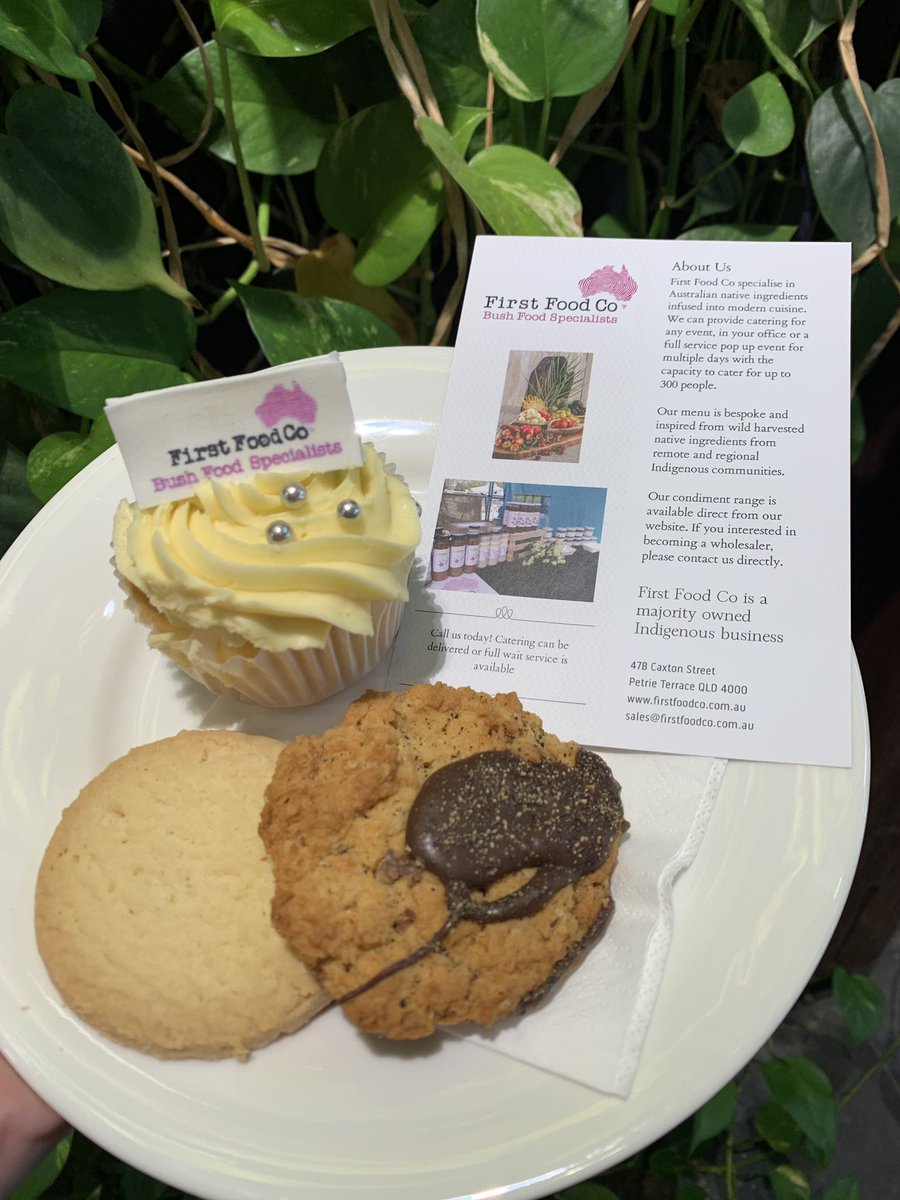In the foreground of the image, a white plate is held against a backdrop of lush greenery, possibly ivy or other shrubbery. The plate, resting on a napkin, carries an assortment of desserts. On the right side sits a cookie that closely resembles an oatmeal raisin, adorned with a generous dollop of melted chocolate. To the left, there's a classic sugar cookie, simple yet inviting. Crowning these treats is a visually appealing cupcake with meticulously swirled yellow frosting, accented by three small silver beads. The cupcake proudly displays a tag reading "First Food Company, Bush Food Specialists," hinting at the company’s Australian roots. A flyer is partially visible, draped over the right side of the plate, further detailing the brand "First Food Company, Bush Food Specialists," and featuring a black silhouette of the Australian continent. The flyer includes the company's address at 478 Caxton Street, Petrie Terrace, Old 4000, along with additional marketing material and contact information. The setting suggests an advertisement, likely for social media, aimed at showcasing these delectable baked goods from an indigenous-owned Australian business.